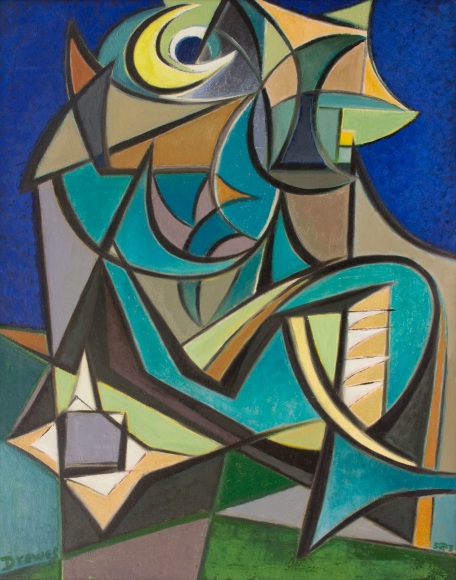This abstract painting, done in a style reminiscent of Picasso, showcases a myriad of geometric shapes and colors on a dark blue background, suggesting a night sky. Dominated by deep blues and punctuated with shades of teal, turquoise, mustard, bright yellow, and greens, the composition features a striking yellow crescent moon in the upper section. Central geometric shapes in earthy tones, such as tans and browns, are interwoven with swirls of light blue, mauve, and white. The bottom section of the painting uses green tones, evoking the sense of grass or a garden, while a distinctive brown triangle hints at forms resembling a bird's beak. A purple square to the left could be reminiscent of a seat. Intricate elements, like an eyeball-like shape in the top left, add intrigue to the piece. The painting is signed "d-y-e-w-e-s" in the bottom left corner, presumably by the artist.